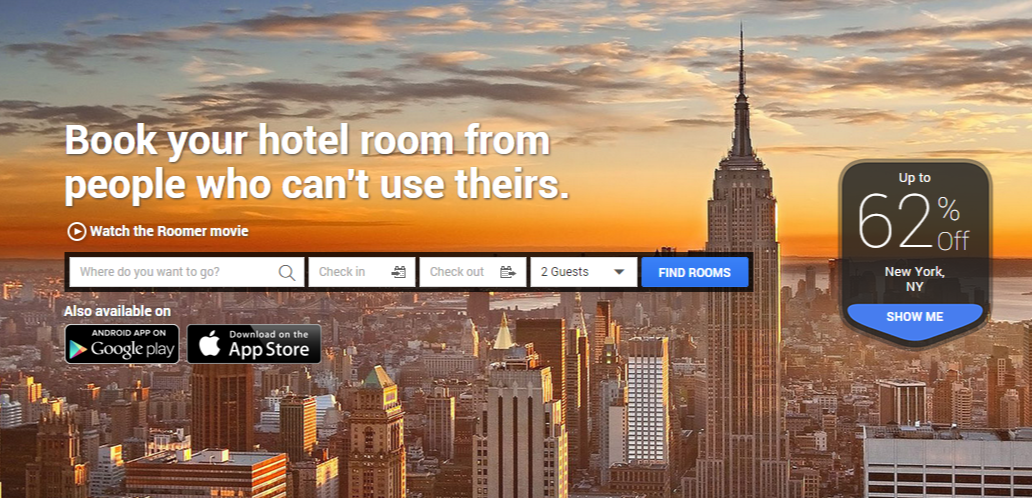*Website Advertisement for a Hotel Booking App*

The website prominently features an advertisement for a hotel booking app called "Globe." The background showcases a stunning cityscape at dusk, with the warm glow of a yellowish sunset illuminating the silhouettes of several tall buildings. The text overlay reads, "Book your hotel from people who can't use theirs." Additional text invites users to "watch the rumor video." 

The user interface provides a seamless booking experience with options to select your destination, check-in and check-out dates, and specify the number of guests. Once the necessary details are entered, visitors can conveniently find available rooms.